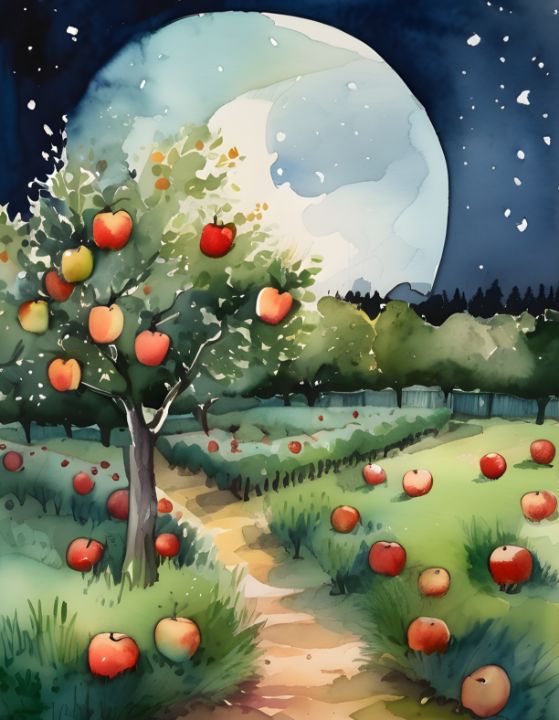This detailed painting depicts an apple orchard at nighttime under an oversized, luminous moon that dominates the sky, almost spanning the entire width of the scene. The sky transitions from black to blue, studded with little white specks and surrounded by dark, stormy clouds. The moon itself shifts in color from white to a light blue, adding to the mysterious ambiance. 

In the foreground, an apple tree with a gray trunk stands prominently to the left of a yellow and brown path that splits into two directions, creating a focal point. Its branches are laden with a mix of red, green, and red-and-green apples, and similar apples are scattered on the grass around the tree, notably on both sides of the path but not on it. Further back, the orchard extends, filled with trees whose tops are green blotches without visible apples, likely due to the distance or the focus of the painting. On the right side of the path, the green floor is dotted with vibrant red apples.

This artwork, possibly a digital design or a watercolor painting, captures a serene and slightly surreal nighttime orchard scene, emphasizing the lush apples and the giant moon's ethereal light.